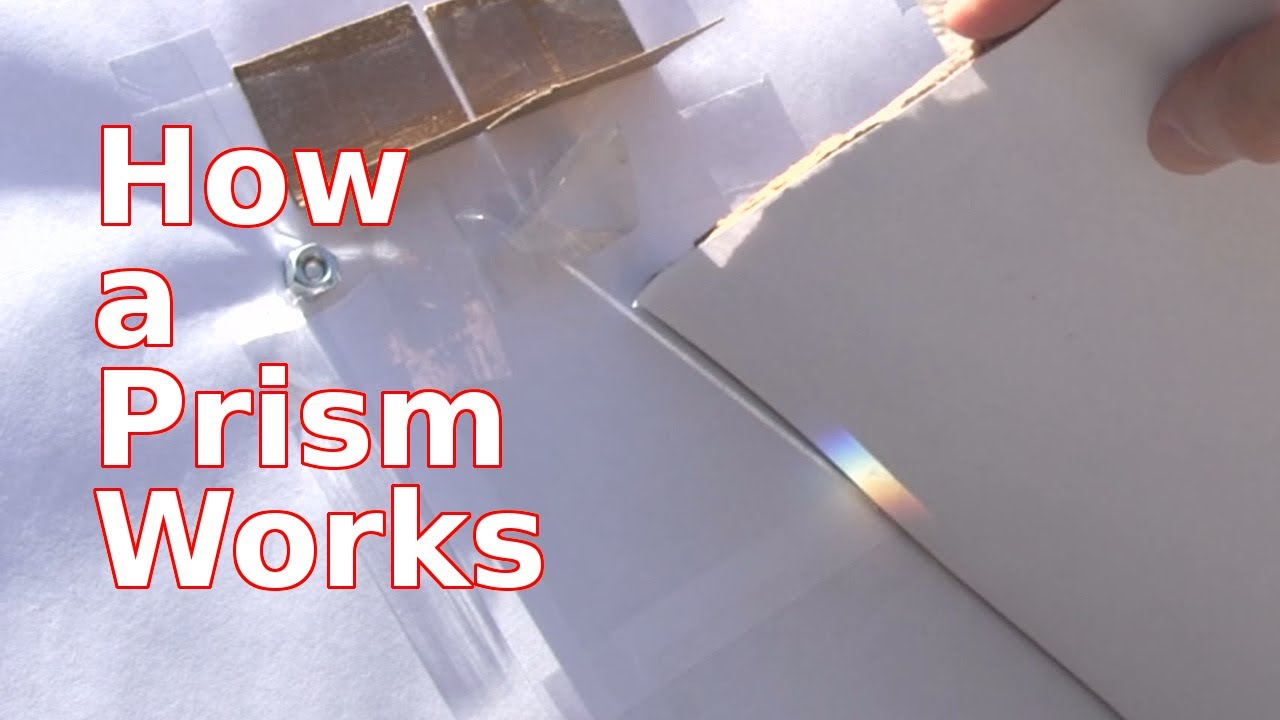The image demonstrates how a prism works, featuring a hand holding a piece of white board or paper. Superimposed on the left side of the image are bold white letters with a red outline, spelling out "how a prism works." In the center, a small, silver gasket is placed between two pieces of cardboard paper, creating a narrow crevice. Sunlight passes through this crevice, interacting with a transparent, triangular prism on the right side, casting a spectrum of rainbow colors, including blue, purple, yellow, pink, and orange, onto the white surface. A person's finger appears in one corner, casting a slight shadow, enhancing the realism and indicating they are outside in direct sunlight, attempting to recreate the prism effect. The setup is partially set against a white background with a paper texture visible on the left.